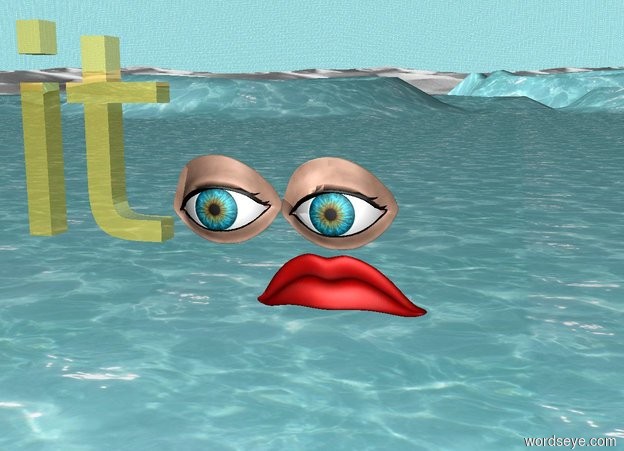This digital animation features a surreal composition dominated by a serene body of bluish-green water with wavy patterns. In the background, a clear blue sky is visible, enhancing the calm yet mystifying ambiance. The water appears to interface with white sand dunes, adding a desert-like feel. Centrally in the image, two human eyes, complete with surrounding skin, float eerily on the water's surface. The eyes have blue irises with black pupils and are looking towards the bottom left of the image, encircled by a slight brown hue. Below the eyes floats a red mouth, adding to the surreal quality. On the left side of the eyes, the word "IT" is written in large yellow letters, partially transparent. In the bottom right corner, the text "wordseye.com" is prominently displayed in white letters. The water interestingly extends into a waterfall towards the top right corner, with some water unusually forming a volcano-like shape in the middle top section of the image.